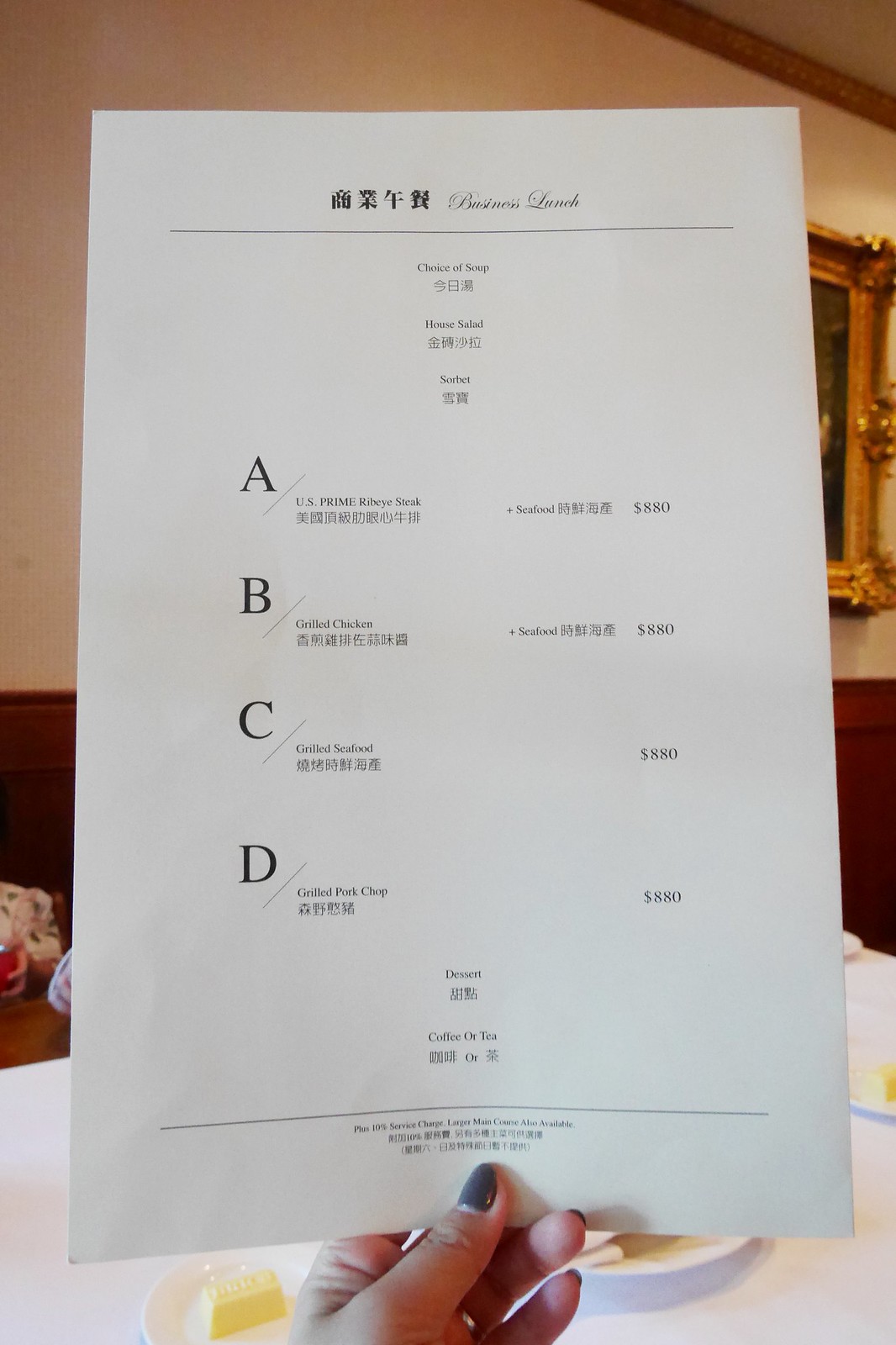The image depicts a woman with a gel manicure, colored gray, holding a plain white menu with her left hand at a restaurant. The menu features Asian script at the top, with the English words "Business Lunch" followed by a list of items and their corresponding Asian characters. The menu offers choices like soup, house salad, and sorbet. It details four main courses: "U.S. Prime Rib Steak" with an option to add seafood for $888, "Grilled Chicken" with the same seafood addition price, "Grilled Seafood" for $880, and "Grilled Pork Chop" also for $880. Below the main courses, the menu mentions "Dessert" and provides a choice of "Coffee or Tea," followed by the restaurant's address. In the background, a white wall is partly covered with a red or wooden panel and features a gold frame.